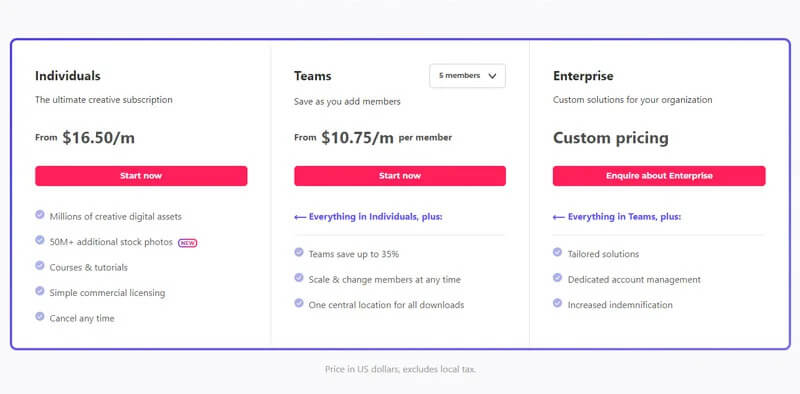The image presents three subscription options for a creative platform:

1. **Individuals**: Marketed as the ultimate creative subscription, this option is priced starting at $16.50 per month. A pink "Start Now" button invites potential subscribers to join. The benefits of this subscription include access to millions of creative digital assets, over 50 million additional stock photos, courses and tutorials, simple commercial licensing, and the freedom to cancel anytime.

2. **Teams**: Positioned to the right of the Individuals option, this plan focuses on cost savings for multiple users, starting at $10.75 per month per user for a default of five members. Similar to the Individuals plan, it features a pink "Start Now" button. This subscription encompasses everything in the Individuals plan plus additional perks such as team savings of up to 35%, the ability to scale and change members at any time, and centralized management for all downloads.

3. **Enterprise**: Tailored for organizational needs, this custom solution offers bespoke pricing. Instead of the "Start Now" button, it features a pink "Inquire About Enterprise" button. It includes everything in the Teams plan, with added benefits such as tailored solutions, dedicated account management, and enhanced indemnification.

Each option is presented with clear headings, detailed benefits, and a prominent call-to-action button, making it easy for potential subscribers to choose the plan that best fits their needs.